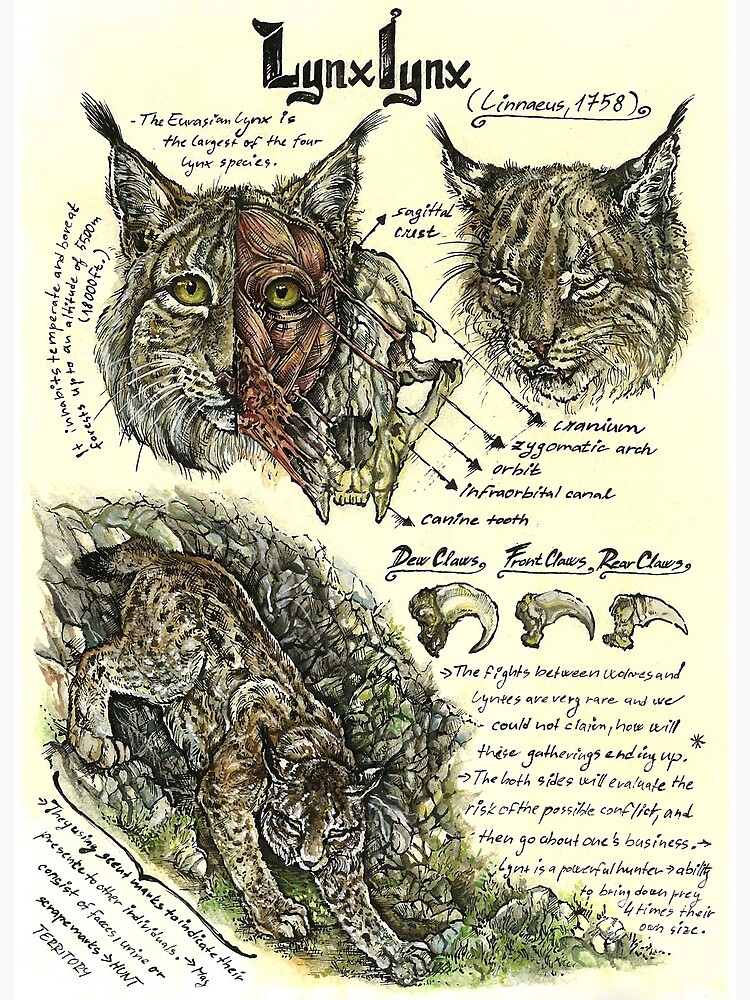The detailed illustration appears to be a pen and ink or color pencil drawing of the Eurasian Lynx (Lynx lynx), resembling a page from a scientific textbook. The rectangular sheet is covered with explanatory handwritten notes and multiple detailed sketches. At the top, the title "Lynx lynx" is repeated, emphasizing the subject. To the left, there is a close-up of the lynx's head; the left side of the head appears normal, while the right side is anatomically dissected to reveal the underlying musculature and skull, with labels pointing to features such as the sagittal crest, cranium, zygomatic arch, orbit, and interorbital canal. 

Adjacent to this, there is another detailed drawing of a fully intact lynx head with downward-cast eyes, labeled with "Alineus 1758" between its pointy ears. Below these head illustrations, in the bottom left corner, is a full-body depiction of a lynx stretching as if emerging from a rocky cave or burrow. Spidery handwriting surrounds it, with more detailed notes describing the lynx's anatomy and behavior, although some text is illegible. 

To the right of these illustrations, there are detailed drawings of the lynx's claws, showcasing the various types: dew claws, front claws, and rear claws, with descriptive labels indicating their different shapes. The entire sheet is a comprehensive study of the lynx, blending artistic skill with scientific precision to present an in-depth look at the wildcat's anatomical features.